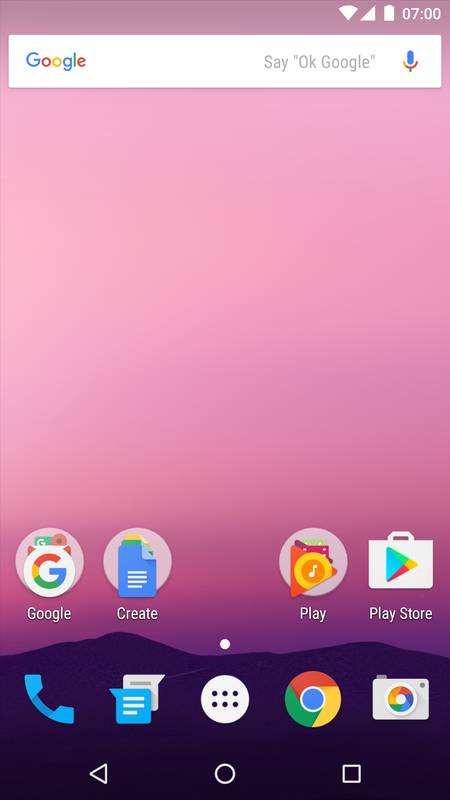The image depicts a smartphone screen with the status bar at the top showing the time as 7:00, along with a white battery icon, a white triangle, and a white signal strength indicator. The main screen is centered around the Google search widget, which has the word "Google" in its iconic blue, red, yellow, and green lettering, followed by the prompt "Say 'OK Google'" and a microphone icon.

Below the search bar is a circular Google icon with the letter "G" in Google colors. Adjacent to it, there are several app icons including:

- A "Create" button represented by folder icons stacked in blue, green, and yellow.
- A Play button that's predominantly yellow with a red triangle inset.
- The Google Play Store icon featuring blue, green, yellow, and red colors.
- A Phone app icon in blue.
- A Texting app icon in blue and white.

Centered at the bottom is a circle with six dots, indicative of the app drawer.

Along the bottom edge of the screen, there are three navigation buttons: a white back arrow, a white circle (home button), and a white square (recent apps button). The lower section of the display screen features a dark blue background that transitions to a pinkish color towards the top.